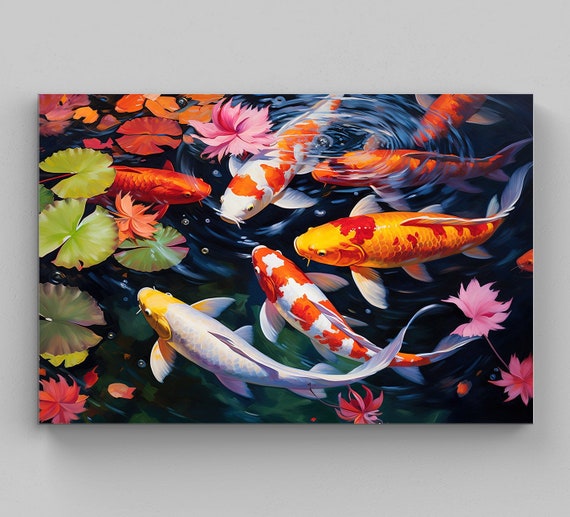This is a vibrant and detailed painting of a koi pond on a canvas, displayed against a gray wall. The artwork portrays seven colorful koi fish, each distinct in its appearance. Among them, there are fish that are white with red spots, orange with red markings, one that is entirely gold with red blotches, and another that is predominantly white with yellow or gold around its face. The fish are depicted swirling near the water's surface, creating ripples and small bubbles that add to the aquatic motion. Surrounding the koi are numerous lily pads and flowers in bright, lively colors including pink, red, orange, and green, which enhance the overall vibrancy of the scene. The water is clear, giving an aerial view of the serene yet dynamic pond environment, accentuated with lush green leaves and resplendent flowers, possibly lilies. The painting is rectangular and rich in detail, capturing the tranquil beauty and vivid colors of the koi and their habitat.